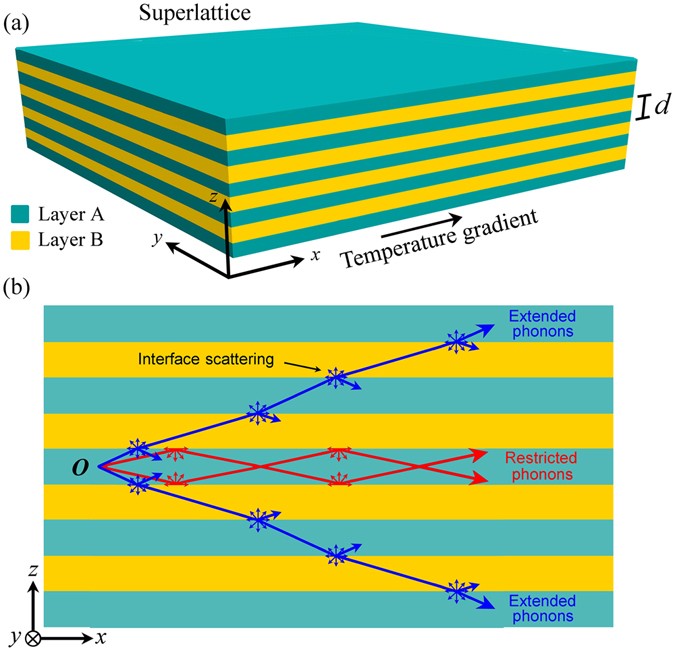The image depicts a detailed graphical representation of a superlattice structure labeled under "A" and "B". In "A", the superlattice is presented as a three-dimensional rectangular diagram consisting of alternating layers of aqua blue and yellow, each labeled as layer A and layer B, respectively. This pattern repeats four times resulting in nine distinct layers. Various arrows mark the edges of this structure, indicating the X, Y, and Z axes and portraying a temperature gradient.

The "B" representation provides a two-dimensional side view of the superlattice, clearly illustrating nine alternating lines of aqua blue and yellow. The diagram includes labels such as "interface scattering" and details the behavior of phonons: with blue arrows signifying "extended phonons" at the top and bottom and red arrows representing "restricted phonons" across the middle. The combination of these views helps to convey the composition and phonon behavior within the superlattice structure.